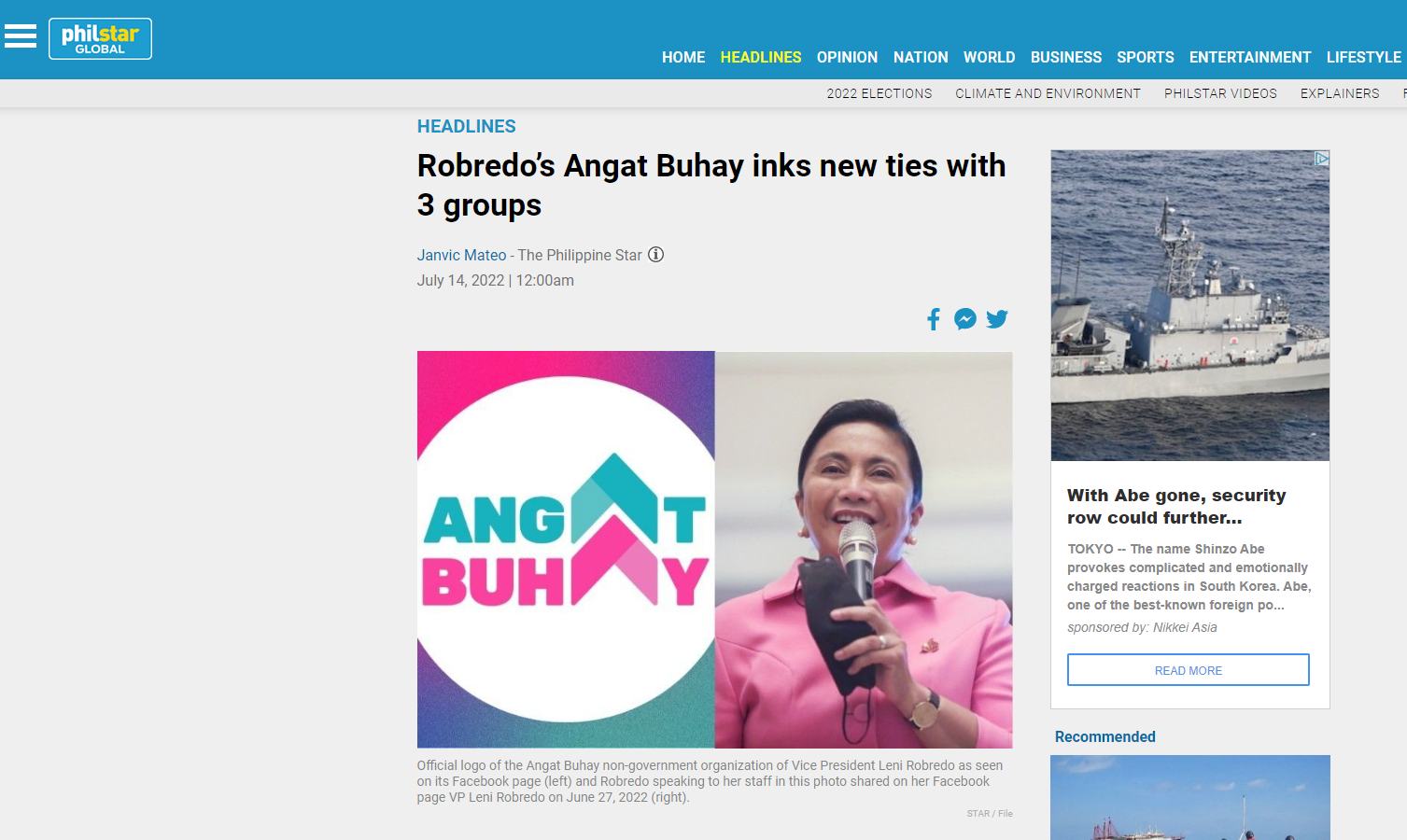In this rectangular screenshot, we're viewing a detailed section from the Phil Star Global website. At the top, a teal banner prominently displays navigational white text listing various sections of the site: "Phil Star Global," "Home," "Headlines," "Opinion," "Nation," "World," "Business," "Sports," "Entertainment," "Lifestyle," "2022 Elections," "Climate and Environment," "Phil Star Videos," and "Explainers."

Beneath the header, bold, black text features the headline: "Robredo's Angat Buhay Inks New Ties with Three Groups" by Janvic Mateo, followed by The Philippine Star and the date: July 14, 2022.

In the main body of the image, a woman is holding a microphone, speaking passionately. Underneath her, a descriptive paragraph elaborates further: "Official logo of the Angat Buhay Non-Government Organization of Vice President Leni Robredo as seen on its Facebook page and Robredo speaking to her staff in this photo shared on her Facebook page, VP Leni Robredo on June 27, 2022."

The image encapsulates a pivotal announcement by VP Leni Robredo, underscoring her NGO's ongoing initiatives and collaborations.